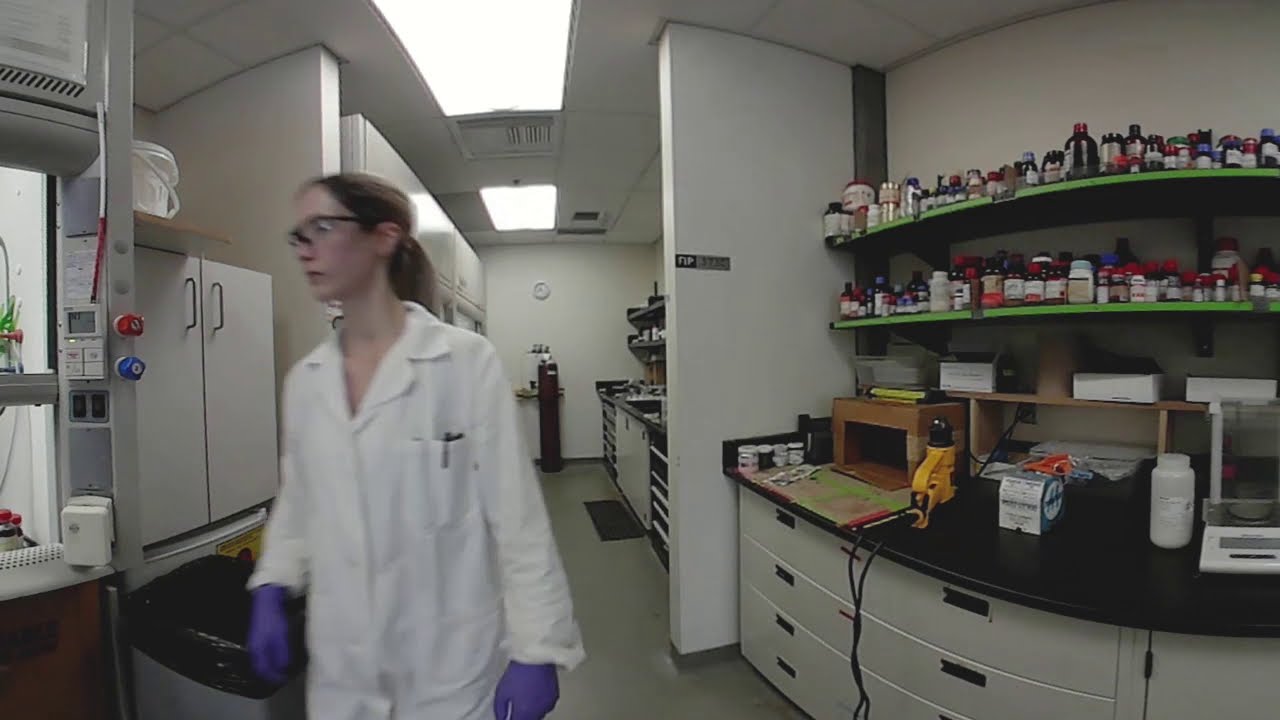In the image, a female scientist or pharmacist is seen in a laboratory or pharmacy testing room. She has long blonde-brown hair tied into a ponytail and is wearing a white lab coat, purple nitrile gloves, and safety goggles with a darker frame at the top. There is a pen visible in her left pocket. Surrounding her are multiple shelves filled with dozens of bottles of various shapes and colors, including brown, red, white, green, and blue. To her right, there is a black countertop with a yellow object on it, backed by green shelves stocked with more medication bottles. A cabinet with two handles and a trash can with a black bag are also situated to her right. Additional lab instruments, a scale, and other standard lab tools are visible throughout the setting, including a red and blue knob and a corded yellow object. The overall scene is a well-equipped, typical laboratory environment.